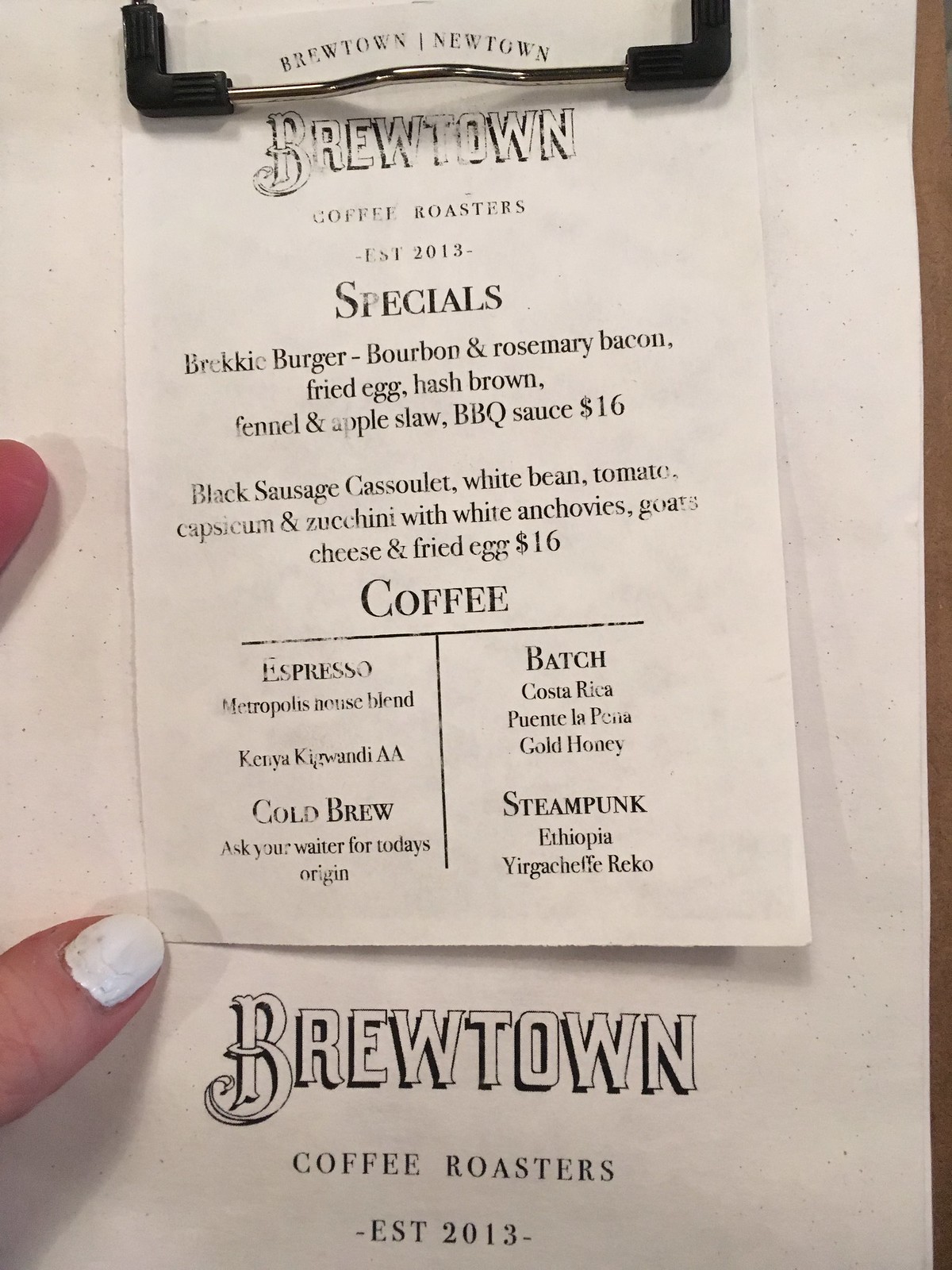The image captures a clipboard with a single sheet of paper clipped to it, featuring the detailed menu of Brewtown Coffee Roasters, established in 2013. Overlaid on the main sheet is a smaller paper, though its contents aren't clear. The focal point includes two fingers holding the clipboard, one adorned with poorly maintained white nail polish.

The menu prominently lists two special breakfast items. The first is a Brekkie Burger, a savory combination of Bourbon and Rosemary Bacon, Fried Egg, Hash Brown, Fennel and Apple Slaw, and Barbecue Sauce, priced at $16. The second special is the Black Sausage Cassoulet, which includes White Beans, Tomato, Capsicum, Zucchini, White Anchovies, Goat Cheese, and a Fried Egg, also for $16.

In addition to the food specials, the menu offers detailed descriptions of the coffee selections. It mentions Espresso brewed with the Metropolis Blend and a Cold Brew made from Kenya AA beans, though the origin details are advised to be confirmed with the waiter. Another coffee option listed is a batch brew made from Costa Rican Gold Honey beans. Lastly, the menu includes Steampunk brewed coffee featuring Ethiopian Yirgacheffe Reku beans.

The text appears to be faint and partially illegible, indicating a less than optimal print job.